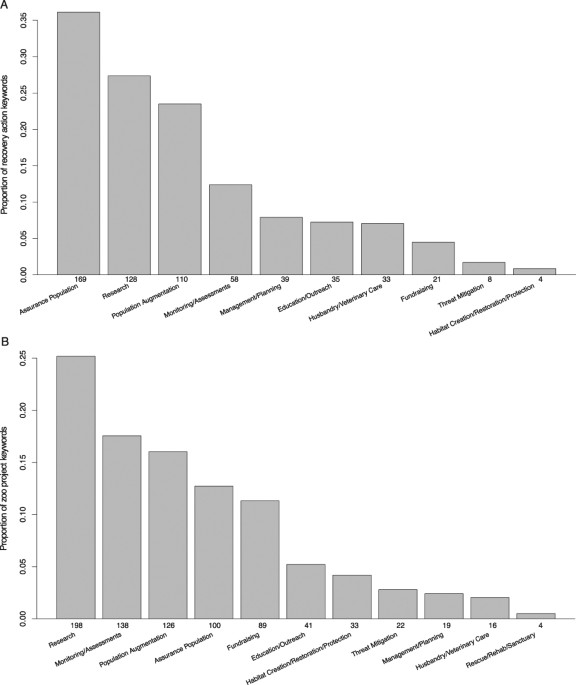The image features two bar graphs labeled "Graph A" and "Graph B" against a solid white background. Both graphs measure proportions, with the vertical axis detailing these proportions and the horizontal axis specifying different keywords. Graph A is titled "Proportion of Recovery Action Keywords" and includes categories such as assurance population, research, population augmentation, monitoring, assessments, management, planning, education, outreach, husbandry, veterinary care, fundraising, threat mitigation, habitat creation, restoration, protection. Graph B, labeled "Proportion of Zoo Project Keywords," lists keywords such as research, monitoring, assessments, population augmentation, assurance population, fundraising, education, outreach, habitat creation, restoration, protection, threat mitigation, management, planning, husbandry, veterinary care, rescue, rehab, sanctuary. The bars are gray and vary in height to indicate the proportion levels, with both graphs having increments from 0.00 to 0.25 on their vertical axes.